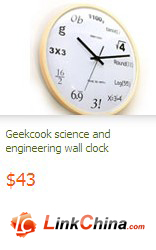Displayed against a white background, this ad features an image of a light beige-framed wall clock with a minimalistic, thin tan border. The clock's face is white, adorned with black hands for hours, minutes, and seconds. Rather than conventional numbers, the clock has unique symbols: 12 reads "1100", 3 is the square root of 4, 6 shows "3!", 8 depicts "16 ÷ 2", 9 presents "3 × 3", 10 is a "G", and 11 shows "OB". Below the clock, the text "Geek Cook Science and Engineering Wall Clock" appears in green letters, accompanied by a price tag of "$43" in red. Adjacent to this detailing, a red icon displays the initials "LC", followed by "linkchina.com" with alternating red and black letters.